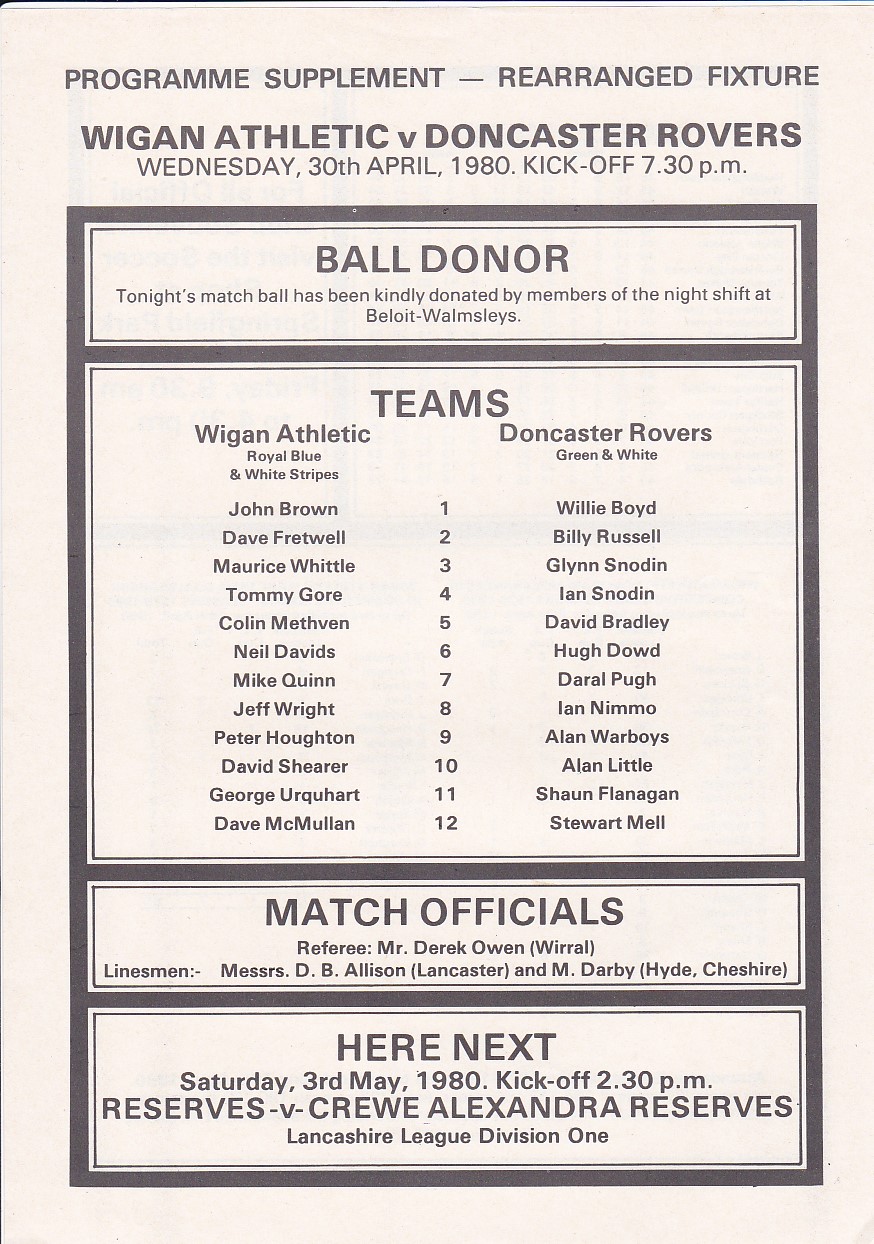The image depicts a weathered ivory white program supplement announcing a rearranged fixture between Wigan Athletic and Doncaster Rovers, set for Wednesday, April 30, 1980, with a kickoff at 7:30 p.m. The supplement opens with the title "Program Supplement - Rearranged Fixture," followed by the bold headline "Wigan Athletic v. Doncaster Rovers." The text, bordered by a black frame, details that the match ball for the evening has been generously donated by the members of the night shift at Beloit Walmsley's. 

Further down, under the heading "Teams," the roster lists the players for both teams. Wigan Athletic's squad includes John Brown, Dave Fretwell, Maurice Whittle, Tom Gore, Colin Methen, Neil Davids, Mike Quinn, Jeff Wright, Peter Houghton, David Shearer, George Uckerhart, and Dave McMullen, clad in royal blue and white stripes. Doncaster Rovers' lineup, in green and white, mentions Merlee Boyd and Billy Russell, among others.

The section titled "Match Officials" lists the referee, Mr. Derek Owen, and the linesmen. The final part of the supplement promotes an upcoming match: "Here Next: Saturday, 3rd May 1980, kickoff, 2.30 p.m. Reserves v. Crewe Alexandra Reserves, Lancashire League Division I."